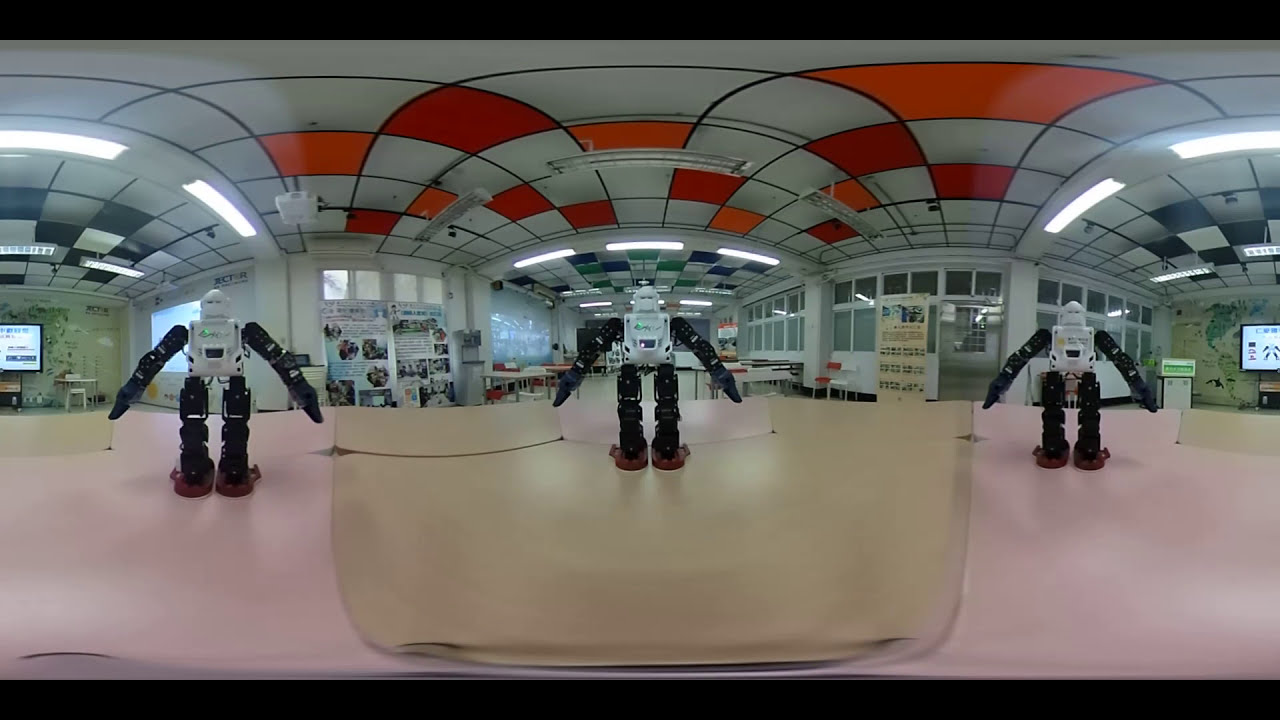This image depicts an intriguing indoor scene featuring three identical robots, each resembling miniature action figures. These robots are arranged in a horizontal line across the center of the room. Each robot boasts a distinctive design with black arms and legs, a white torso, and a white head. The room features an eye-catching ceiling composed of various geometric shapes, with sections shaded in orange and light red. At the back of the room, large windows, doorways, a collection of unreadable signs, and big TV screens are situated. The floor below the robots is predominantly tan in the middle, transitioning to pink along the sides. The setting appears to be a specialized shop, possibly a body shop dedicated to creating action figures. The 360-degree camera view or a framing effect adds a unique perspective, emphasizing the central robot from the back, enhancing the overall depth and complexity of the scene.